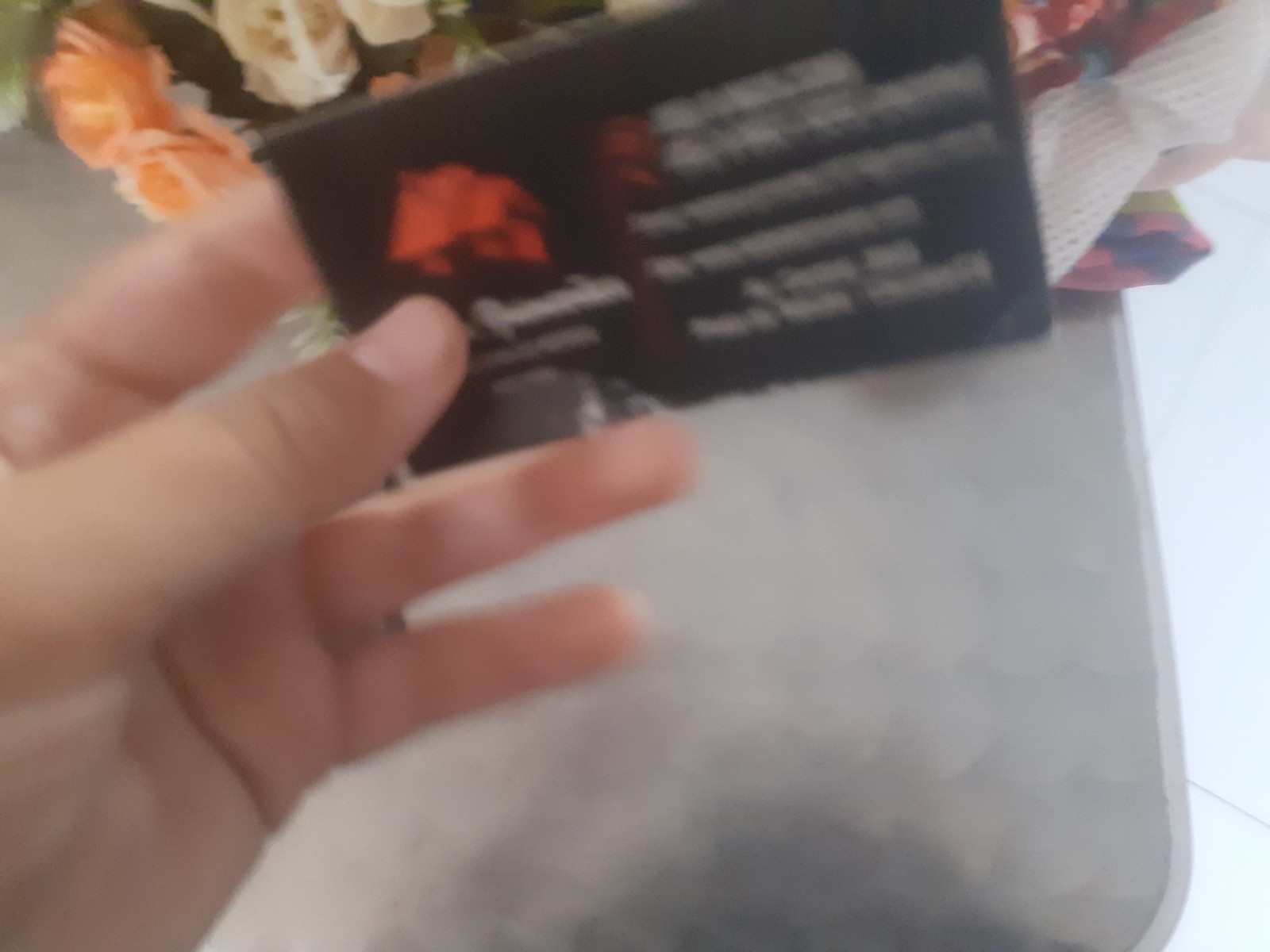A left hand is prominently featured on the left side of the image, partially visible. The hand appears to be holding a black card, which has a house design but looks blurry. The background is adorned with what seems to be flowers, adding a touch of nature to the scene. At the bottom, there is a gray mat providing a neutral base. On the right side of the image, there is a white object, though its details are not clear.